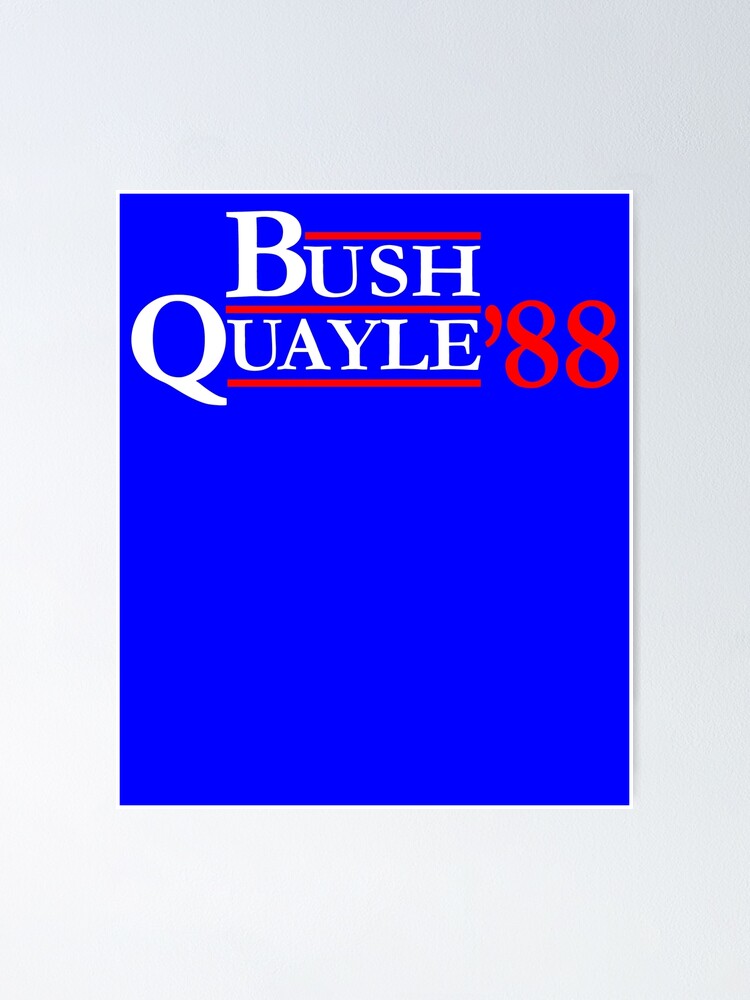The image depicts a rectangular billboard-style sign from the 1988 Bush-Quayle presidential campaign. The background is primarily a solid blue rectangle, bordered by a thin white line. This blue section occupies the center of the image, which itself lies on a light gray background. Positioned at the top of the blue rectangle, in large, bright white text, are the names "Bush" and "Quayle," separated by a pair of red horizontal lines; one above and one below the text. Following these names is "'88," written in bold red. The text occupies roughly the top third of the blue rectangle, leaving a significant blank blue space beneath it. This minimalist design emphasizes the Bush-Quayle 1988 logo, with its patriotic color scheme and stark simplicity.